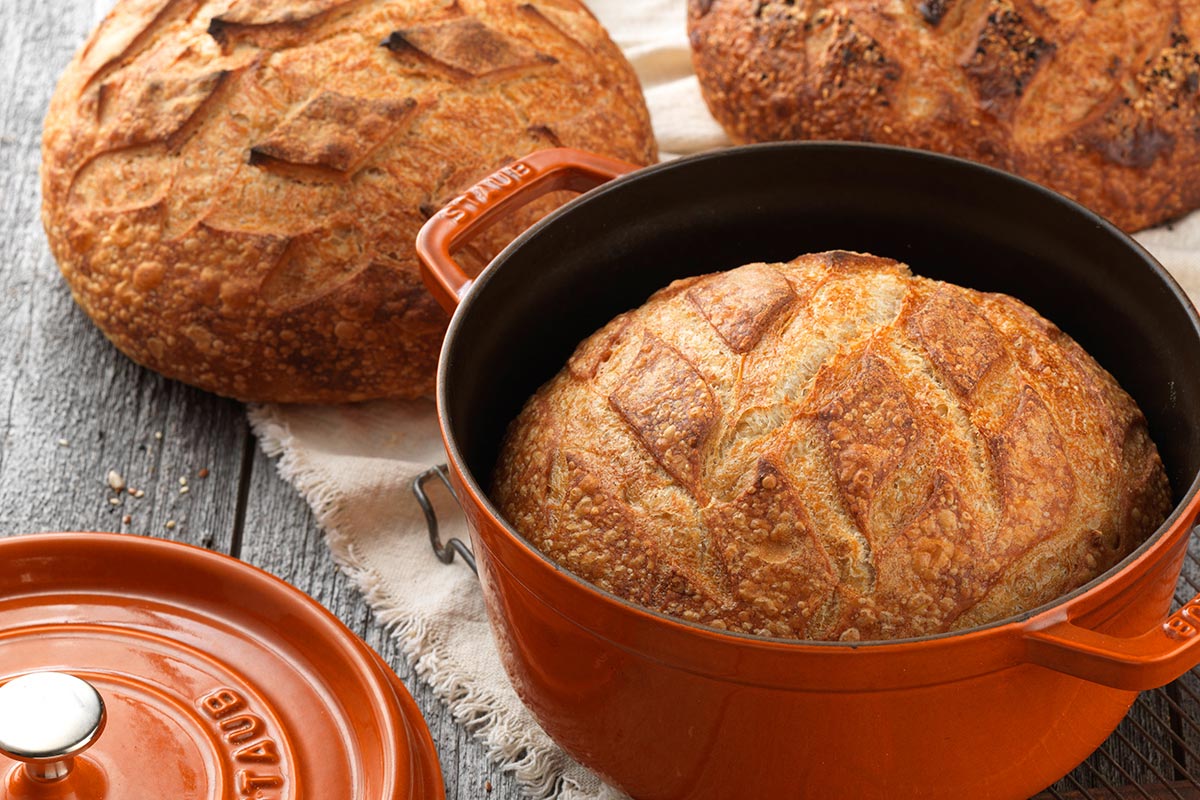The image is a detailed photograph featuring an arrangement of sourdough bread. At the center right, there's a pot with a black interior and a red (or orange) exterior—referred to as a casserole dish—containing an oval-shaped loaf of sourdough bread. This bread appears to be brown with some cracks on its surface. Engraved text "STAUB" is visible on both the pot's handle and its lid, which rests beside the pot in the bottom left corner of the image.

Above and to the left of the red pot, on a white cloth (which could be a tablecloth or napkin), there are two more loaves of sourdough bread. One loaf is fully visible in the upper left corner, sharing the same oval shape and brown color as the bread in the pot. The second loaf is only partially visible, with just a portion sticking out on the upper right side of the image.

All the items—the red pot with its bread, the two additional loaves, and the white cloth—are placed on a table. The table appears to be wooden, with descriptions varying between a rough dark gray and a shade of brown in color. The collective scene is coherent and aesthetically pleasing, highlighting the rustic charm of freshly baked sourdough bread.